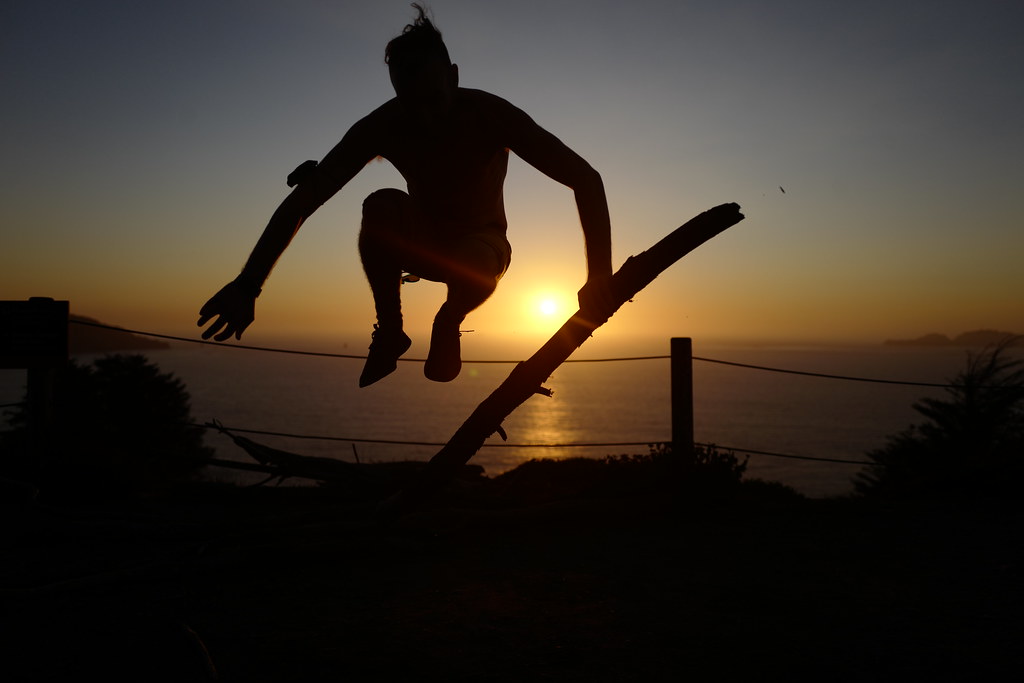The photograph captures a striking outdoor scene at sunset, featuring a silhouetted person in mid-air. The person is leaping while holding onto a twisted tree trunk or rod with their left hand, with their right hand extended outward. The individual is clad in shoes and shorts, and appears to either be wearing a tank top or be shirtless, which is suggested by the visible hair under their arms. The sky transitions from a deep blue at the top to a golden hue near the horizon, where the sun is setting, casting an orange tint over the ocean. The sun's reflection shimmers on the still waters below. The foreground is entirely black, filled with the dark shapes of plants. To the right of the person is another upright post, adding an element of balance to the composition. The overall mood is serene and silhouetted, with a mix of natural elements enhancing the beauty of the moment.